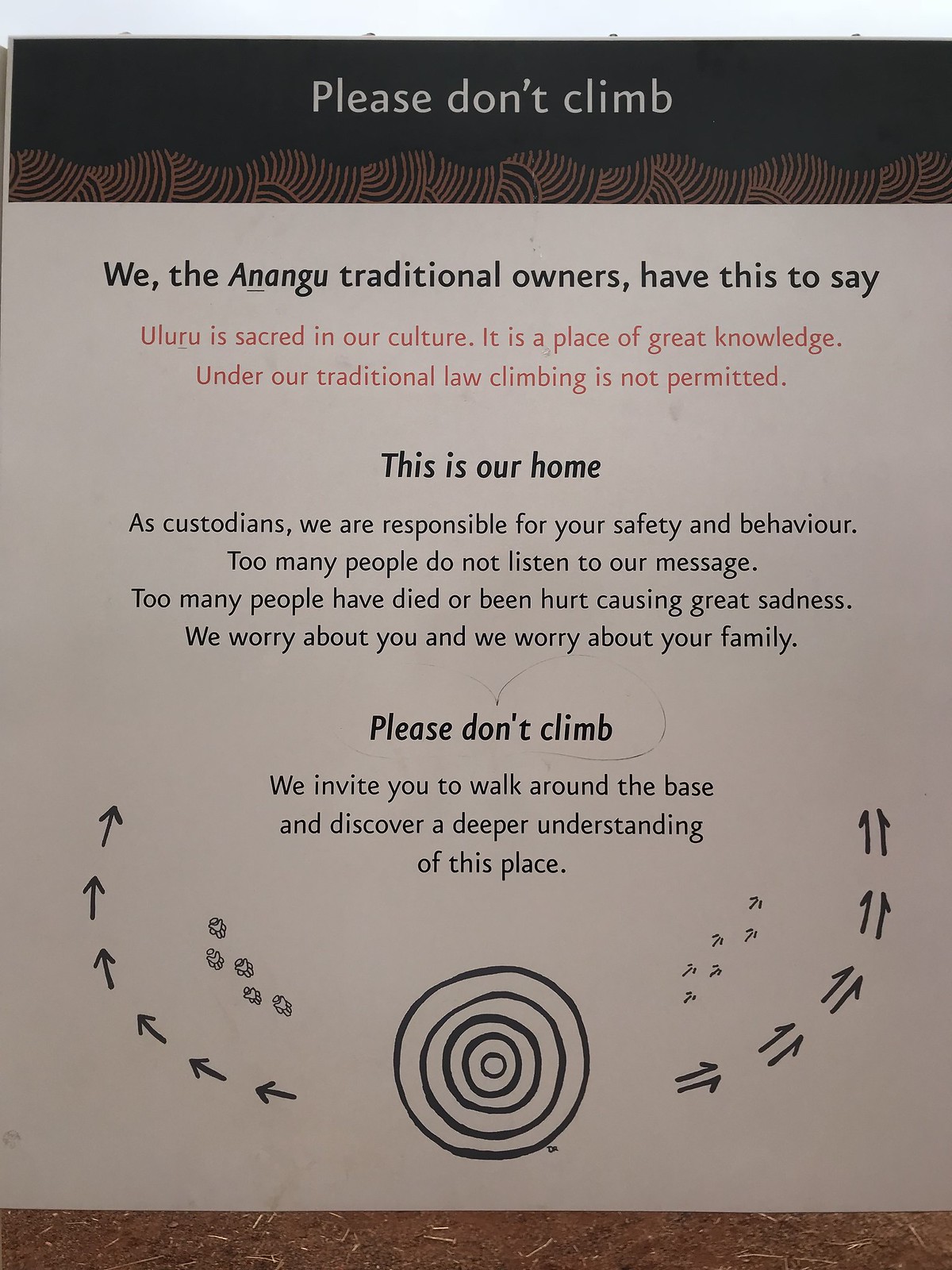This image is a detailed and color photograph of a portrait-oriented poster that describes important cultural rules at a facility. The poster features a black horizontal band at the top with bold white lettering that reads, "Please Don't Climb." Below this, a light cream-colored main section bears a message from the Anangu traditional owners in black type: "We, the Anangu traditional owners, have this to say." This is followed by impactful red text: "Uluru is sacred in our culture. It is a place of great knowledge. Under our traditional law, climbing is not permitted." Beneath this, black text continues: "This is our home. As custodians, we are responsible for your safety and behavior. Too many people do not listen to our message. Too many people have died or been hurt, causing great sadness. We worry about you and we worry about your family. Please don't climb." The message closes with an invitation: "We invite you to walk around the base and discover a deeper understanding of this place." At the bottom of the poster, a hand-drawn circular design is depicted, featuring concentric circles with arrows pointing left and right. Surrounding the circles are images of paw prints and footprints, symbolizing movement and exploration. The style of the poster is photographic realism, and it includes small brown designs resembling hills for a decorative touch.